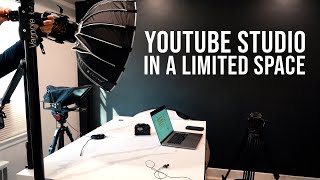The image depicts a compact and well-equipped YouTube studio. Dominating the background is a black screen bearing white text that reads "YouTube Studio in a limited space." The room is filled with various pieces of filming equipment arranged closely, indicating a small, cramped setup. On the left is a prominent studio light, partially obscured, and a tripod stands nearby without any equipment mounted on it. A white desk occupies the center of the scene, cluttered with a small laptop (possibly a Macintosh), a camera, a microphone, a remote control, and various black wires and USB cables. The laptop is powered on, though its display contents are indiscernible from the image. Additionally, multiple cameras on tripods are situated around the space—one closer on the right and one further back. Colors in the space are predominantly neutral, including shades of gray, white, off-white, black, and silver, with sparse hints of orange and blue. Although one mention included hands adjusting a light, no discernible people or signs of life or activity are visible, reinforcing the notion of an inactive yet meticulously arranged recording setup.